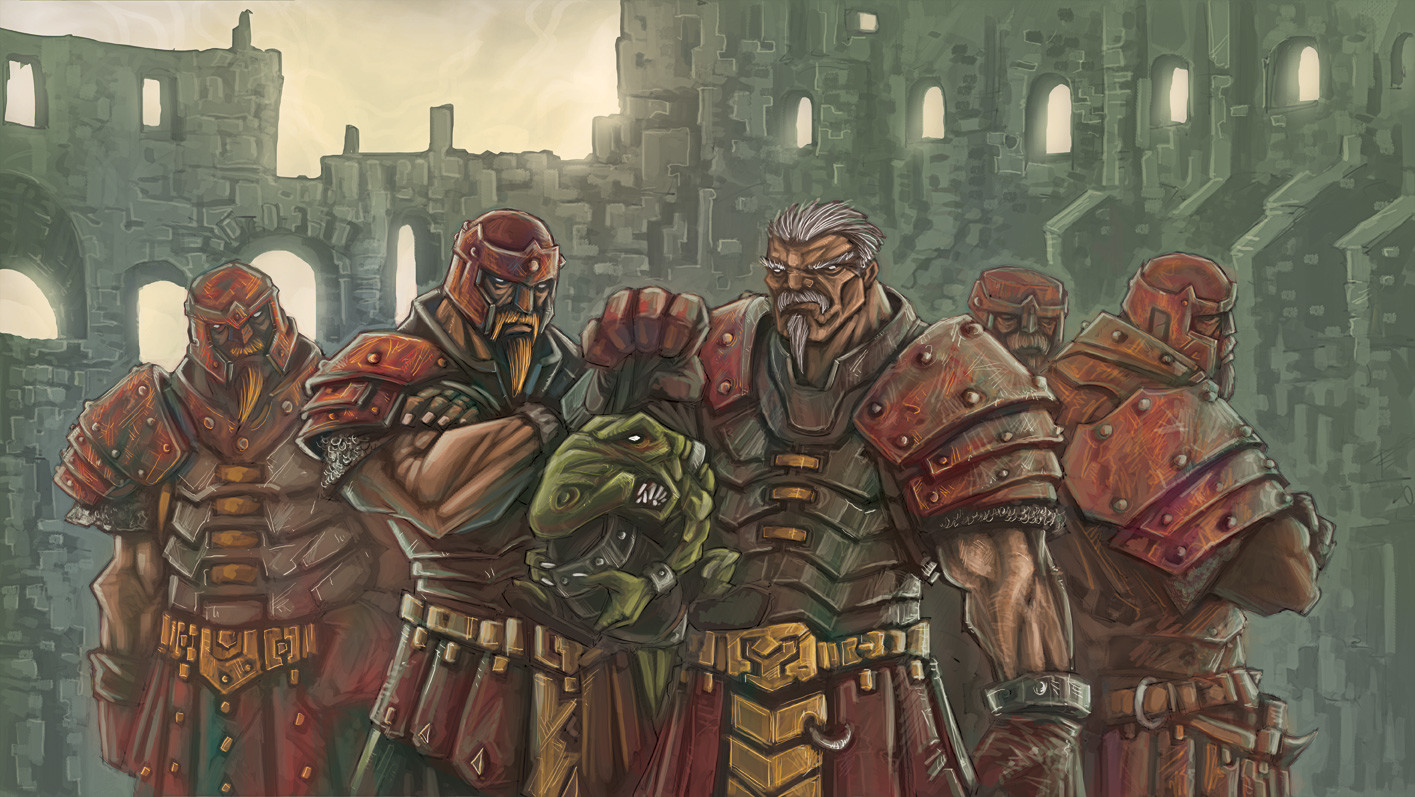This is a highly detailed computer-animated image of five knights, depicted with exaggerated, robust muscular builds. Their thick armor, adorned with shoulder plates and metal belts, accentuates their formidable presence. Each knight sports a medieval look, complete with armored helmets and various protective gear, including ear pieces and gloves. The man in the center stands out with his helmet removed, revealing his gray hair, bushy eyebrows, mustache, and goatee, coupled with an angry expression. He holds a green, frog-faced helmet in his hand. Among the knights, the one to his left crosses his arms and wears an orange helmet, complemented by matching facial hair. Their reddish outfits add a striking contrast to the scene, which is set against a backdrop of a green-brick palace under a tannish-beige sky, evoking a medieval ambiance.